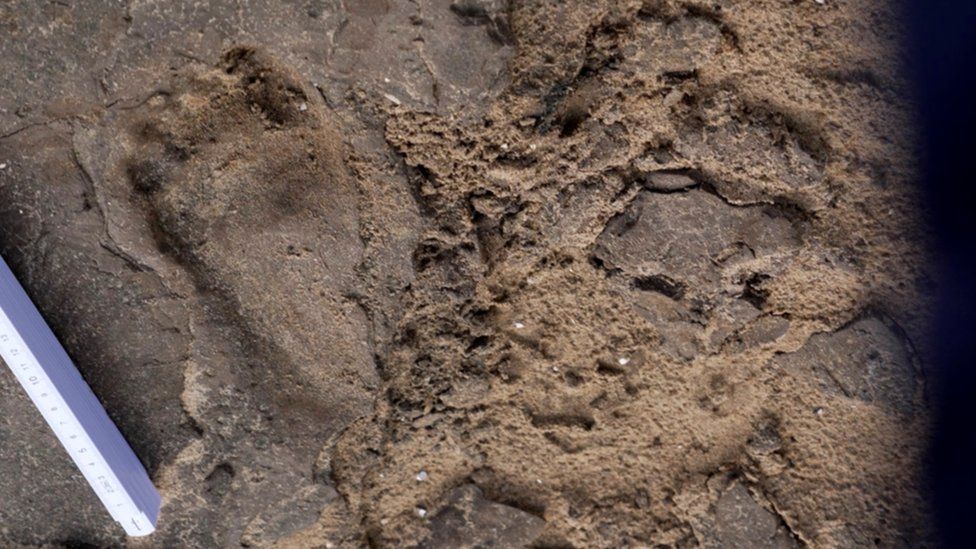The image presents a close-up view of a rocky and muddy surface, displaying various shades of brown and gray. Dominating the left side of the photograph is an unusual human-like footprint, which instead of being an indentation, intriguingly bulges outwards, suggesting it may have been created from below the surface. The footprint itself is large and triangular, with a wide toe area narrowing towards the heel. Adjacent to the footprint, there's a ruler featuring a blue bottom stripe and white top section with black numbers, likely included to measure the footprint's length. The overall setting appears rugged and might be archeological in nature, indicating the possible discovery of an ancient or fossilized footprint amidst dark brown, lighter brown, and grayish rocky terrain.